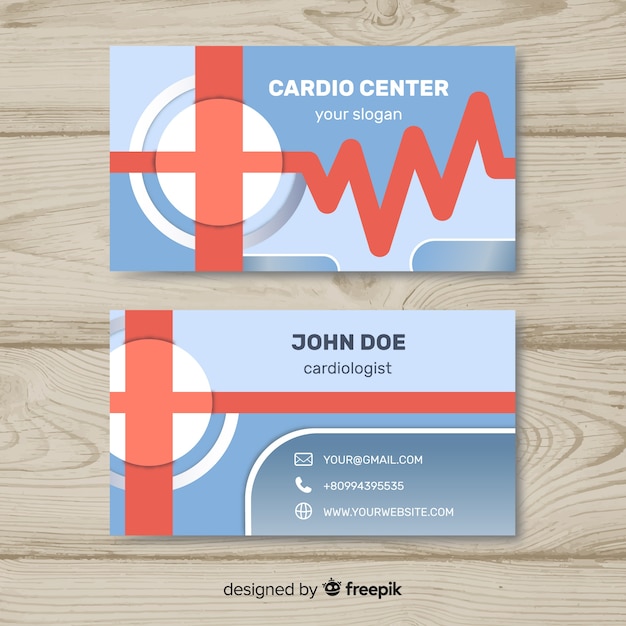The image is an advertisement for business cards set against a light wooden background made up of four horizontal planks, showcasing the wood grain. The top card has a light blue background with a prominent red cross on the left that transitions into an EKG line with peaks and valleys in red. The text "Cardio Center" is written in white, followed by a placeholder "Your Slogan" below it. A white circle with a border enhances the design on the left side. The bottom card also features a light blue section at the top, with the name "John Doe" in bold black text, followed by "Cardiologist" in thinner black text. It includes a vertical red stripe on the far left and a horizontal thin red stripe above the midsection. Below this stripe, icons for email, telephone, and website are present with corresponding sample information: "yourgmail.com," "+809-943-9535," and "www.yourwebsite.com." Both cards incorporate shades of light and darker blue. At the very bottom of the image, against the wooden background, the phrase "designed by Freepik" is printed in thin black letters alongside a small crown logo, identifying the design company.